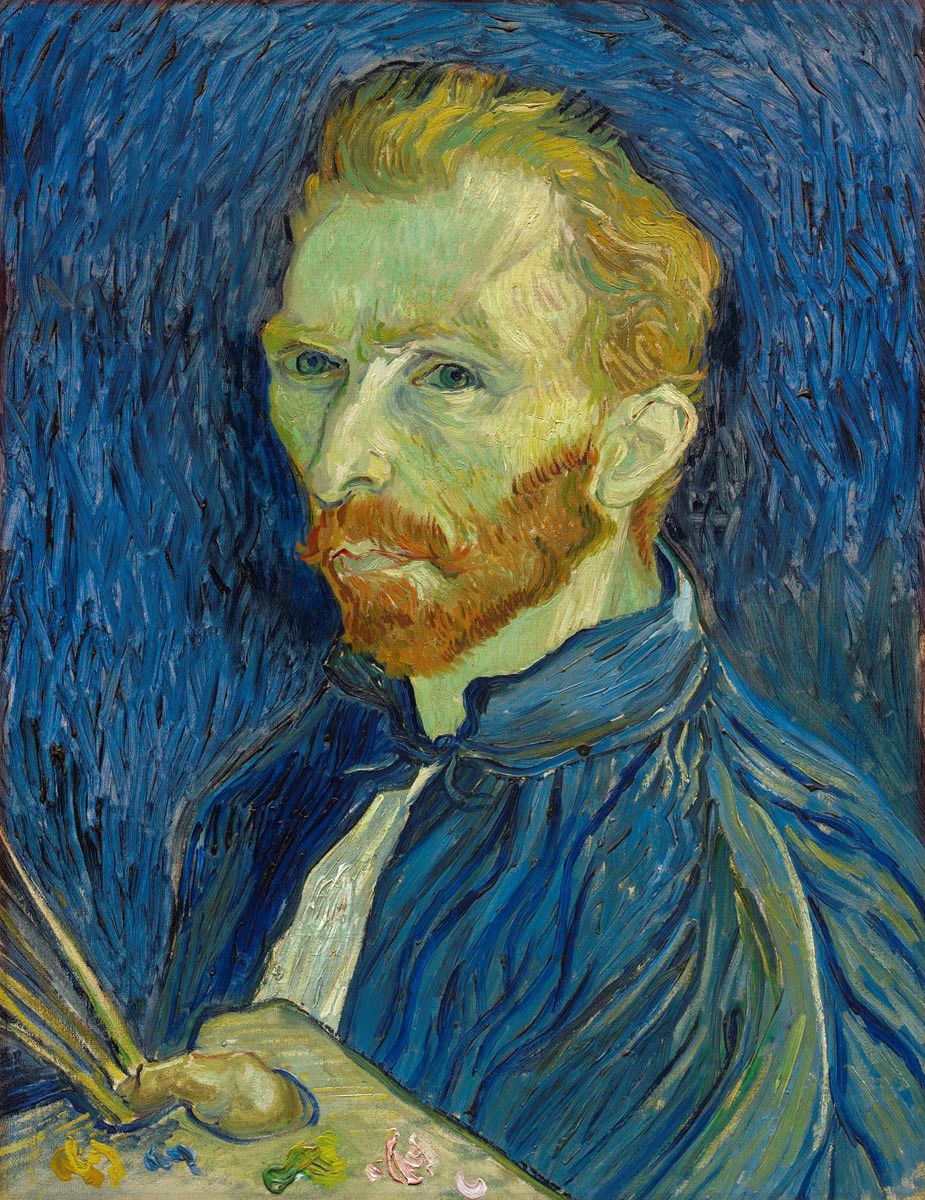This painting depicts a self-portrait of the famous artist Vincent van Gogh. The artist features golden-reddish hair and a full reddish beard. He is seen wearing a blue shirt with a tied collar. In his hand, he holds a painter's palette, which contains various vibrant colors including green, pink, blue, and yellow. The background of the painting is a blue hue with Van Gogh's characteristic spiral strokes, creating an abstract ambiance. The figure looks focused and serious, with a concentrated expression as he holds his painting tools, indicative of his engrossment in the act of creation.